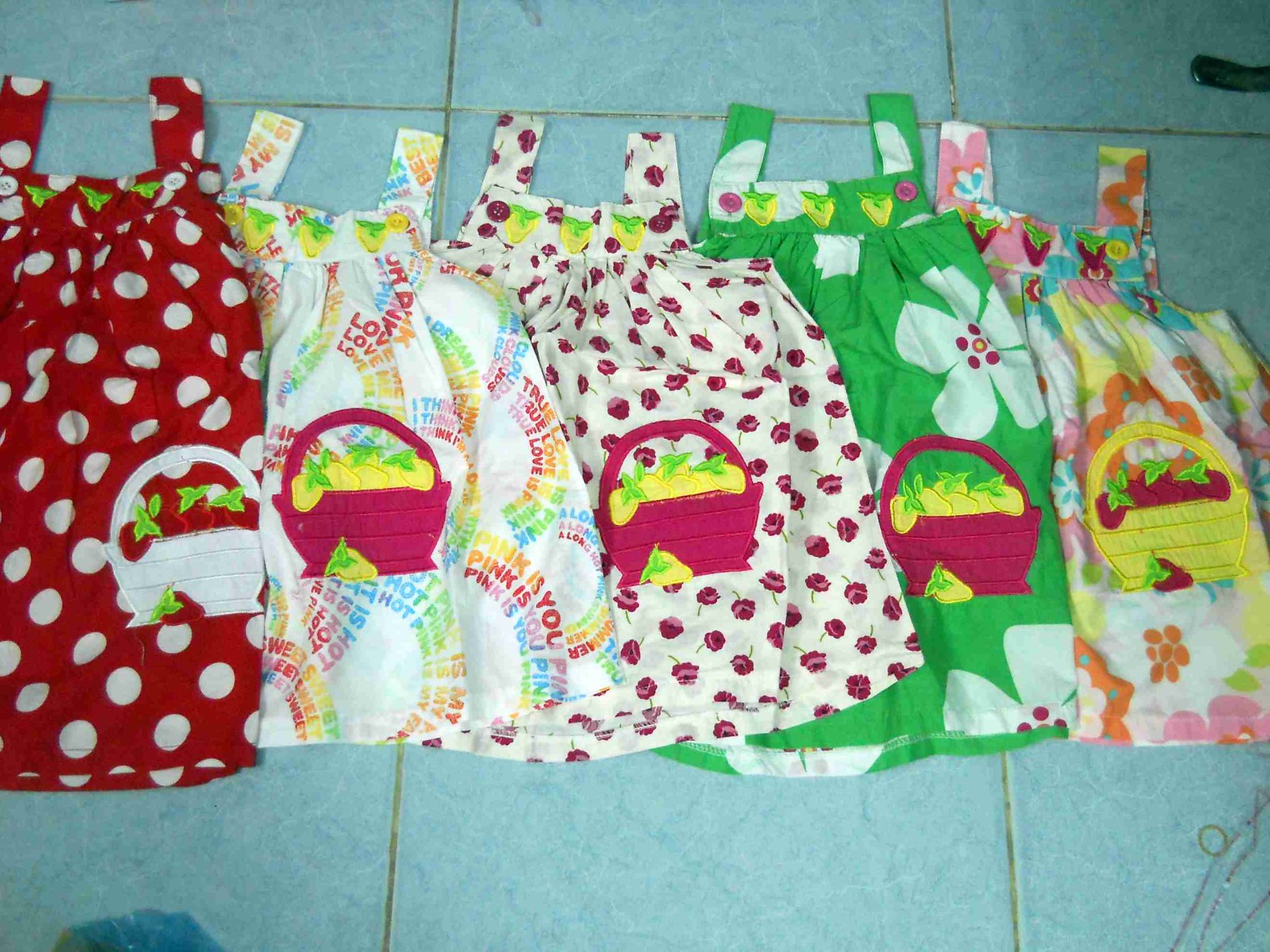The image displays five colorful, sleeveless sundresses for a toddler girl, approximately two years old, laid out side-by-side on an aged, blue tile floor. Each dress, embroidered with a basket of strawberries, shares a similar style and length, extending just above the knees. From left to right: the first dress is red with white polka dots, featuring a white basket of strawberries with green leaves; the second dress has a white background adorned with multicolored lettering and a red basket filled with yellow strawberries; next is a white dress with pink roses and a coordinated pink basket of yellow strawberries; following that, a green dress showcases large hibiscus flowers, paired with a pink basket and yellow strawberries; finally, a multicolored floral dress completes the lineup with a yellow basket containing red strawberries. The dresses show slight overlap in the image, emphasizing their cohesive, handcrafted design.